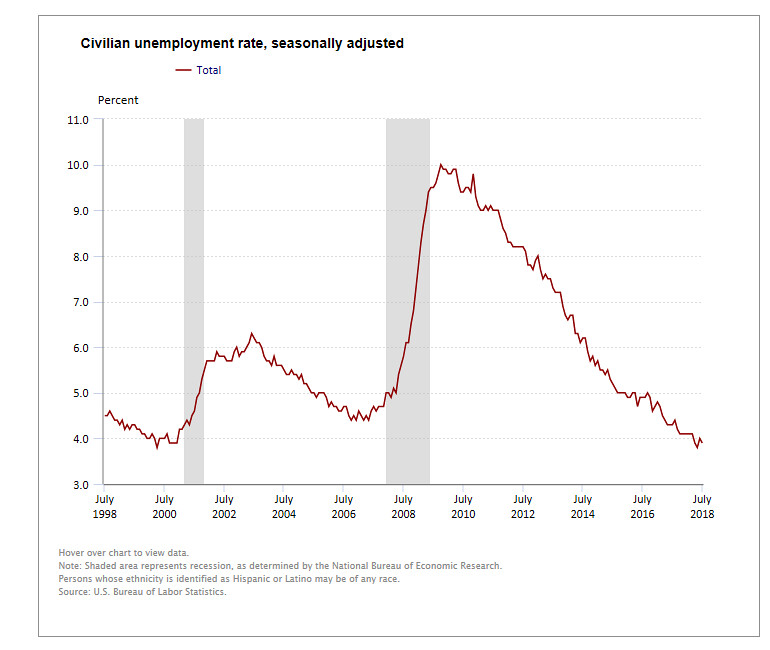This image displays an informative graph illustrating the civilian unemployment rate, seasonally adjusted, over a period from July 1998 to July 2018. The background is white, and the graph prominently features a red, lightning-like line indicating the total unemployment rate. At the top, in black text, it is labeled "Civilian Unemployment Rate Seasonally Adjusted," with "total" in red beside a red line, and "percent" also in black beneath it. 

On the left vertical axis, percentages are marked, ranging from 3.0 at the bottom to 11.0 at the top. On the horizontal axis at the bottom, years are denoted in black, indicating key points such as July 1998, July 2000, July 2002, July 2004, July 2006, July 2008, July 2010, July 2012, July 2014, July 2016, and July 2018. The graph shows notable trends, with a sharp increase in unemployment peaking around July 2010, reaching close to 10.0%, and then a decline through to July 2018.

In the bottom left-hand corner, gray text provides additional information: "Hover over chart to view data. The blue shaded area represents recession as determined by the National Bureau of Economic Research. A person whose ethnicity is identified as Hispanic or Latino may be of any race." The source of the data is the U.S. Bureau of Labor Statistics.